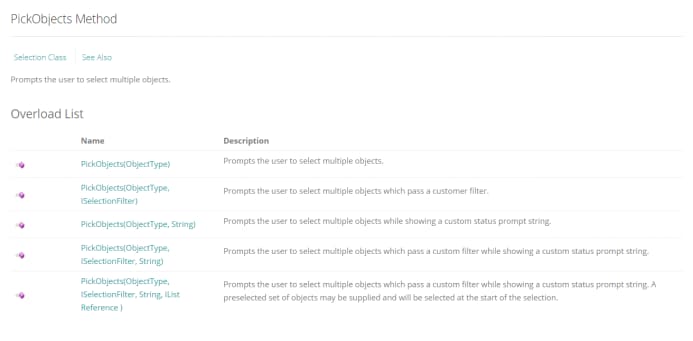A blurry and light screenshot captured in landscape mode from a laptop showcases a software interface. In the upper left corner, the text "Pick Objects Method" is displayed prominently. Below it, underneath a slender gray line, two tabs are visible: "Selection Class" in green on the left, and "See Also" in green on the right. 

Despite the blurry quality, some details beneath these tabs can be discerned. A gray prompt instructs the user to "select multiple objects." Further down, labeled "Overload List," there is a grid comprising three columns and six rows. 

The first column is filled with purple blurs, while the second column, titled "Name," lists various methods: 

1. Pick Objects (Object Type)
2. Pick Objects (Object Type, Selection Filter)
3. Pick Objects (Object Type, String)
4. Pick Objects (Object Type, Selection Filter, String)
5. Pick Objects (Object Types, Selection Filter, String, IList Reference)

The third column, named "Description," contains the corresponding descriptions for these methods:

1. Prompts the user to select multiple objects.
2. Prompts the user to select multiple objects with a custom filter.
3. Prompts the user to select multiple objects.
4. Prompts the user to select multiple objects with a custom filter.
5. Prompts the user to select multiple objects with various filters applied, including a list reference.

Each row in this grid gives a detailed description of different overloads for the "Pick Objects Method," assisting the user in choosing the correct operation based on their specific needs.